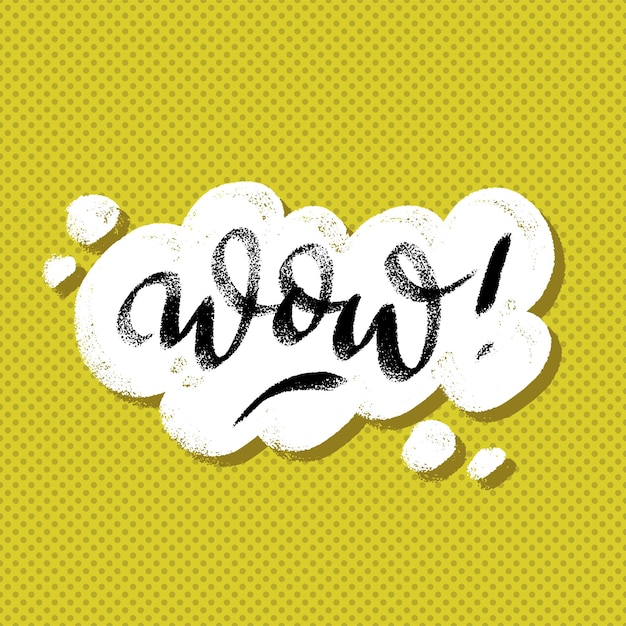This digital illustration features a square format with a vibrant background. The backdrop is a greenish-yellow hue, adorned with small, olive-green polka dots densely packed across the entire space. Overlaid on this lively background is a hand-drawn word bubble in white, exhibiting a chalk or airbrush texture consistent with digital art. Inside the bubble, the word "WOW!" is prominently displayed in black, also in a hand-drawn, airbrushed style, suggesting it was created with a stylus. The word is underlined and ends with an exclamation point, emphasizing the amazement it conveys.